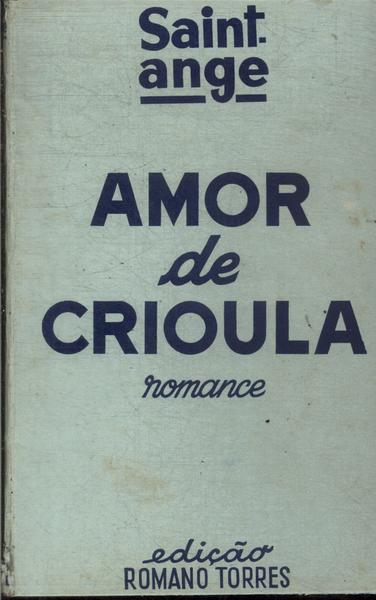The image depicts a worn book cover set against a cream-colored background marred by smudge and dirty spots. At the top, in navy blue lettering, "Saint Ange" is prominently displayed, with "Ange" underlined by a thick blue line that interacts with the letter 'G'. Centrally aligned is the title "AMOR" in bold, uppercase letters, followed by "DE" in a delicate script, and "CRIOULA" again in uppercase. Below this, the word "romance" is elegantly scripted, and after a substantial blank space, "EDICAO" appears in cursive at the bottom, with "Romano Torres" beneath it. The background shows signs of age with stains and a weathered gray tone, while the edges, particularly the bottom and left, are darkened, suggesting the presence of a binding.